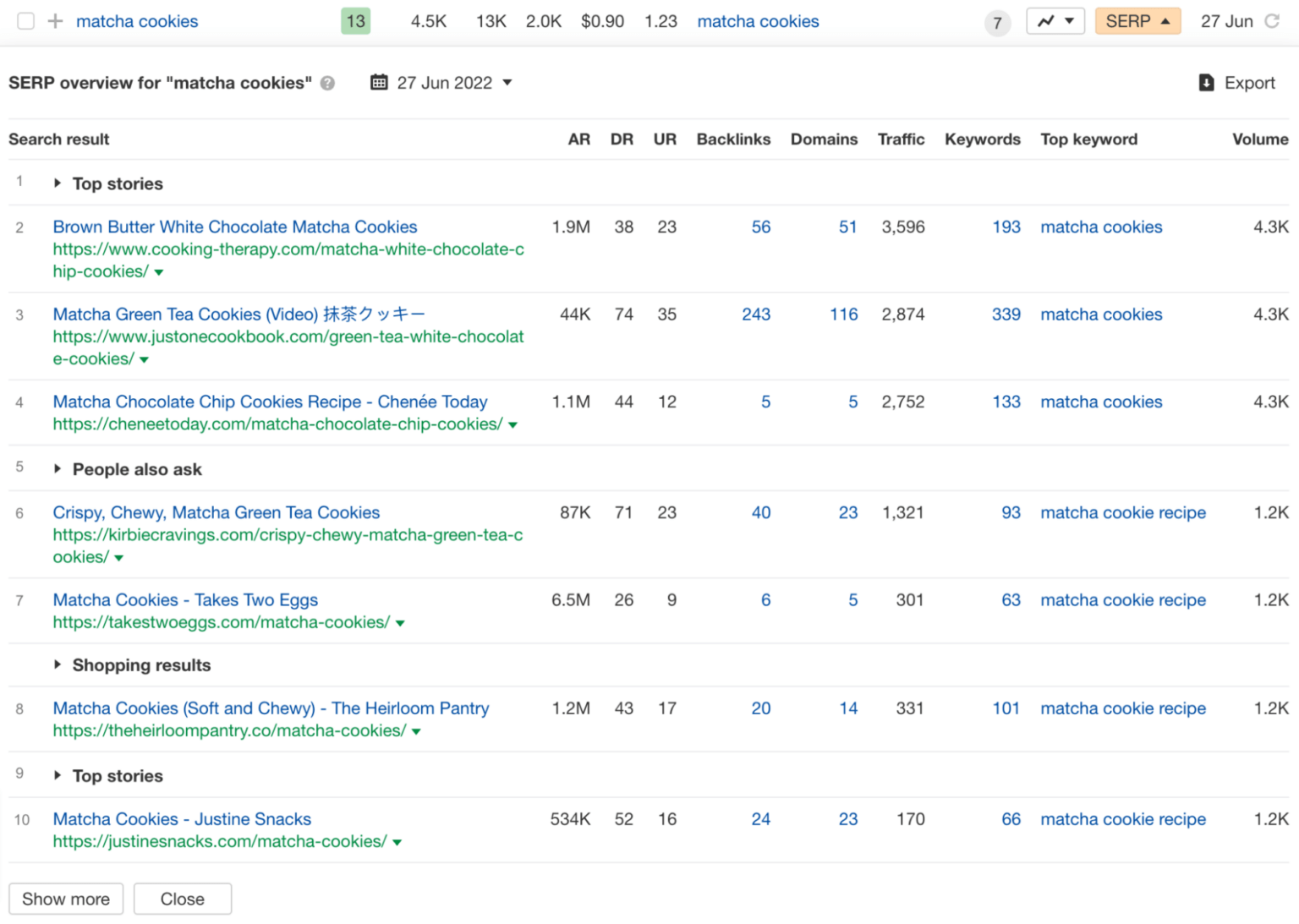In the detailed menu, the header prominently announces "Matcha Cookies" and includes several numerical values: 13, 4.5k, 13k, 2.0k, 90 cents, and 1.23. Additionally, the heading mentions the number 7 and features an emblem for the stock market report with the acronym SERP (Search Engine Results Page) and the date 27 June.

The body of the menu opens with a list of search results titled "Top Stories." The first listing reads "Brown Butter White Chocolate Matcha Cookies" with a corresponding web address that appears as a string of alphanumeric characters: 1.9MAR38DR23UR. This listing also includes the following metrics: bank backlinks (56), domains (51), traffic (3596), keywords (193), with the top keyword being "matcha cookies," and an indication to "buy in" at 43.5.

The next entry is "Matcha Green Tea Cookies Video" which also includes an email address and similar metrics across the page. Another listing, "Matcha Chocolate Chip Cookies Recipe," is attributed to chenaytoday along with a web address.
 
Following these is a section titled "People also ask," containing user questions such as "Crispy Chewy Matcha Green Tea Cookies" with an accompanying web address. Another question mentions that matcha cookies require two eggs, also followed by a web address.

The menu continues with "Shopping results," highlighting "Matcha Cookies Soft and Chewy" from The Heirloom Pantry, accompanied by a web address. Under the "Top Stories" section, "Matcha Cookies Justine Snacks" is listed with its web address. To conclude, there are options to "Show More" or "Close" the list, displayed as buttons.